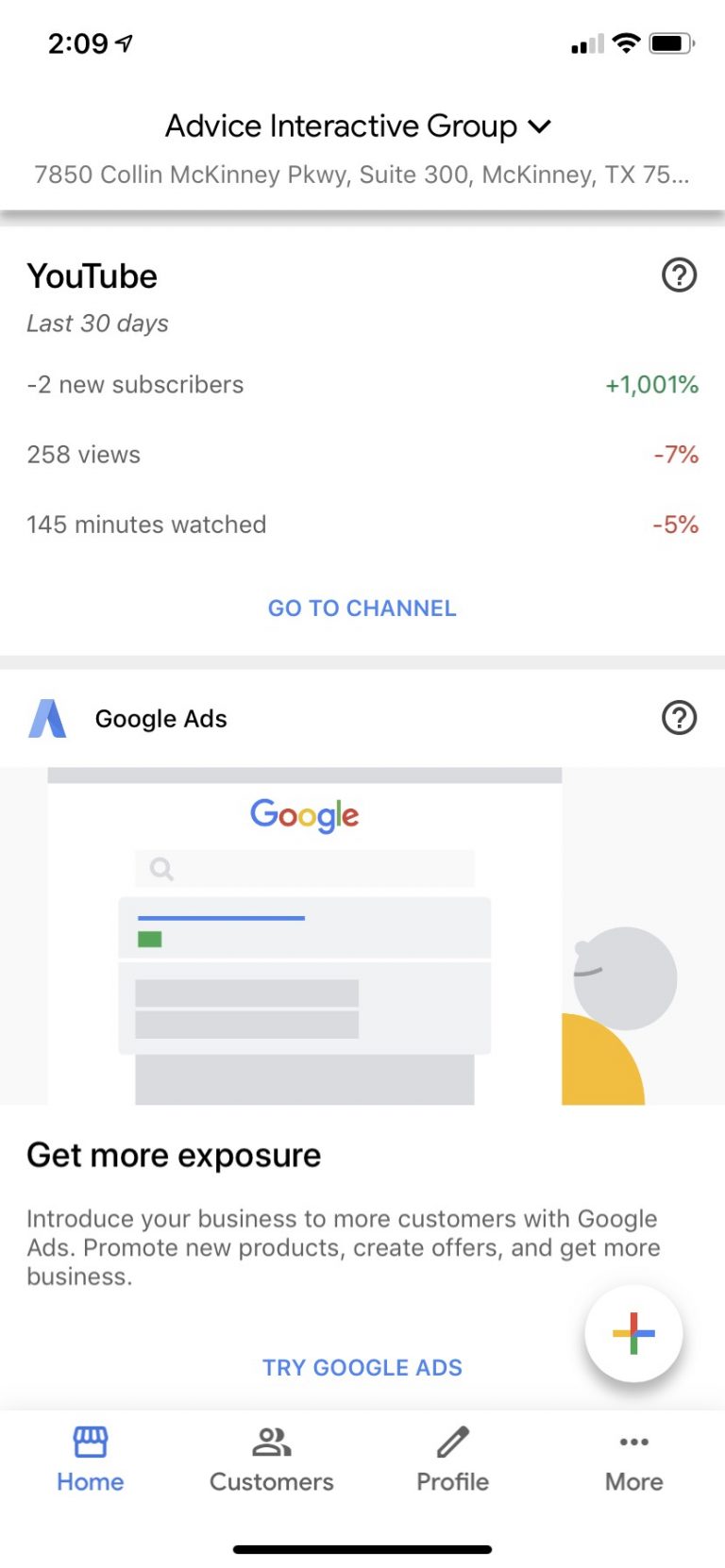The image features a smartphone screen with a white background. At the top of the screen, there is a text header in black that reads "Advice Interactive Group." Below this, the address is provided as "7850 Collin McKinney Parkway, Suite 300, McKinney, TX 75070."

Underneath the address, the left section displays YouTube analytics for the last 30 days, noting "-2 new subscribers," while the right section shows a green increase of "+1.001%." Further down, on the left, there are "258 views," with a red "-7%" indicating a decline. Additionally, there are "145 minutes watched," marked with a red "-5%."

A blue link follows, stating "Go to Channel." Below this, a message reads, "CookieX: We don't have data to finish a [fusion] get more exposure introduce your business for more customers with CookieX promote new products create offers and get more." There’s another blue link below it: "Try New CookieX."

To the right of this message, there is a white button with a plus sign in red, green, yellow, and blue colors. At the bottom, there are four navigation tabs: "Home" on the far left, highlighted in blue, followed by "Customers," "Profile," and "More" on the far right.